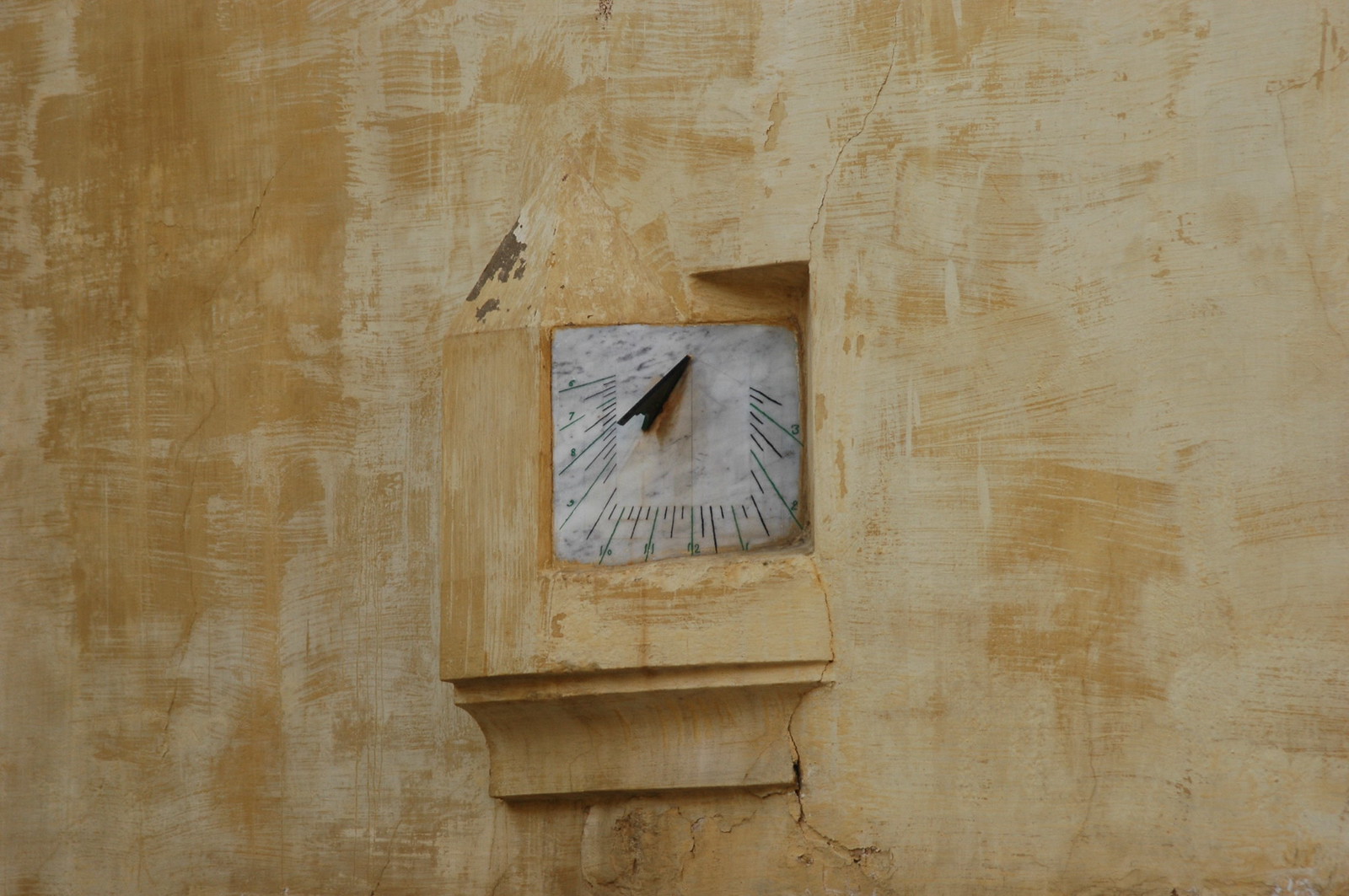This image features a clock embedded in a beige-toned wall, which exhibits a rustic, textured appearance with visible cracks extending upward and downward from the clock. The wall itself is divided into lighter and darker beige hues, contributing to an overall aged and weathered aesthetic. At the center of the frame, the clock face stands prominently, characterized by its whitish color and marked with dark, thin minute and hour hands. The clock's numeral markings display an unusual configuration, spanning from three to nine, with the nine positioned higher than typically expected, giving the entire setup a distorted look. Additionally, the clock hands appear oddly intertwined, contributing to the surreal, almost AI-generated feel of the composition, enhancing the eerie peculiarity of the scene.